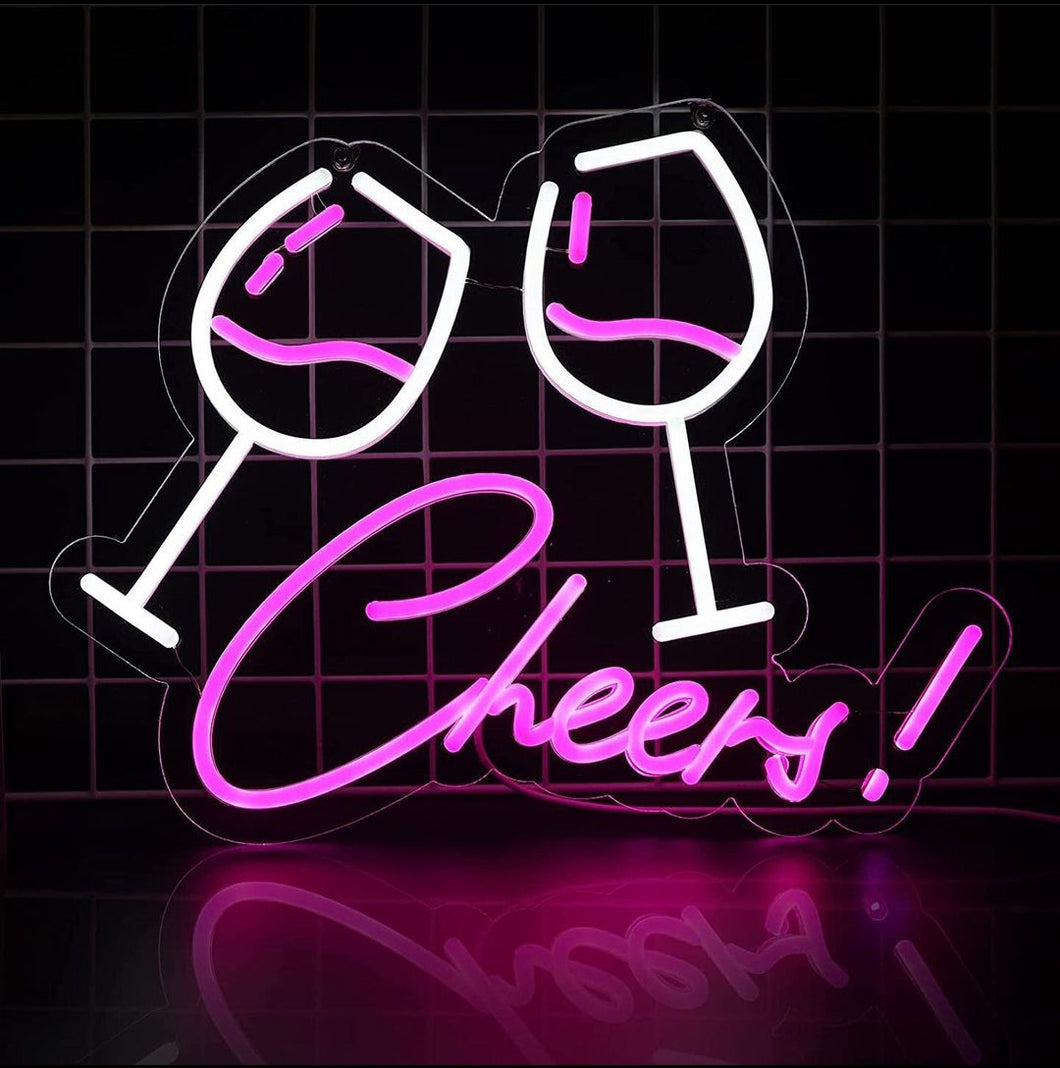The photograph features a vibrant LED neon sign leaning against a white grid wall with a black background. The neon tubes are meticulously bent into the cursive word "cheers!" with a magenta hue, complete with an enthusiastic exclamation mark. Above the word "cheers!", two stylized wine glasses appear to clink together; the glass on the left is slightly more tilted than the one on the right. Both glasses are depicted with a pink liquid inside, and the left glass even shows droplets spilling out, adding a dynamic touch. The neon sign is set in a white acrylic base, adding to its polished look. Below the sign, an extremely shiny surface reflects the entire design, amplifying the vivid colors and festive vibe of the product. The overall staging, including the reflective surface and the grid wall background, suggests a product photo aimed at selling this upbeat and fun electric sign. The contrast between the magenta lettering and pink reflections against the black and white tiled background makes the sign stand out, further enhancing its visual appeal.